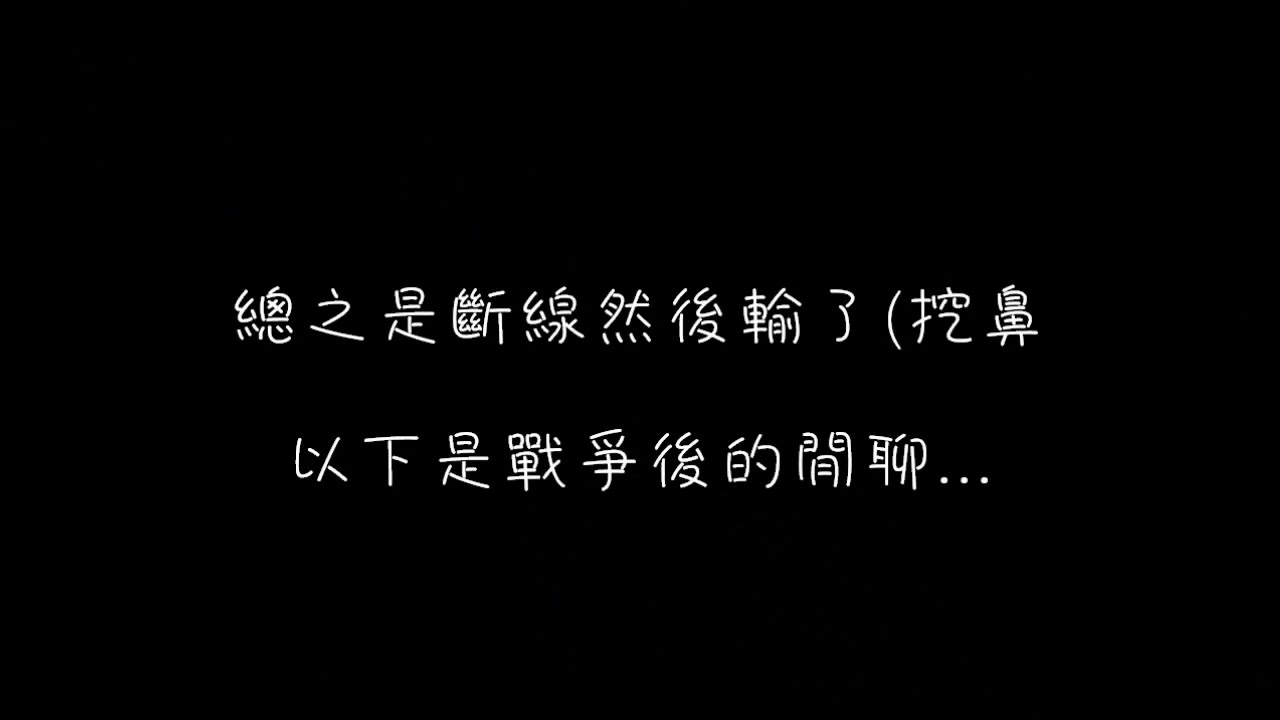The image features a horizontal black rectangular background with two rows of intricate white text, resembling an oriental script, likely Chinese. The top row contains 11 distinct symbols or characters. Notably, the seventh symbol resembles a house, while the eighth looks similar to the numeral three. The second to last symbol on this row appears to be a combination of a plus sign and the number two. The bottom row includes nine smaller, detailed drawings or symbols. The second symbol from the left on this row appears akin to a capital 'F'. The other symbols are abstract, consisting of squiggly lines and shapes, with the last one ending in three dots, creating an ellipsis. The overall script conveys a message translated as "I was disconnected and lost (nose picking)," followed by, "the following is a small talk after the war..."